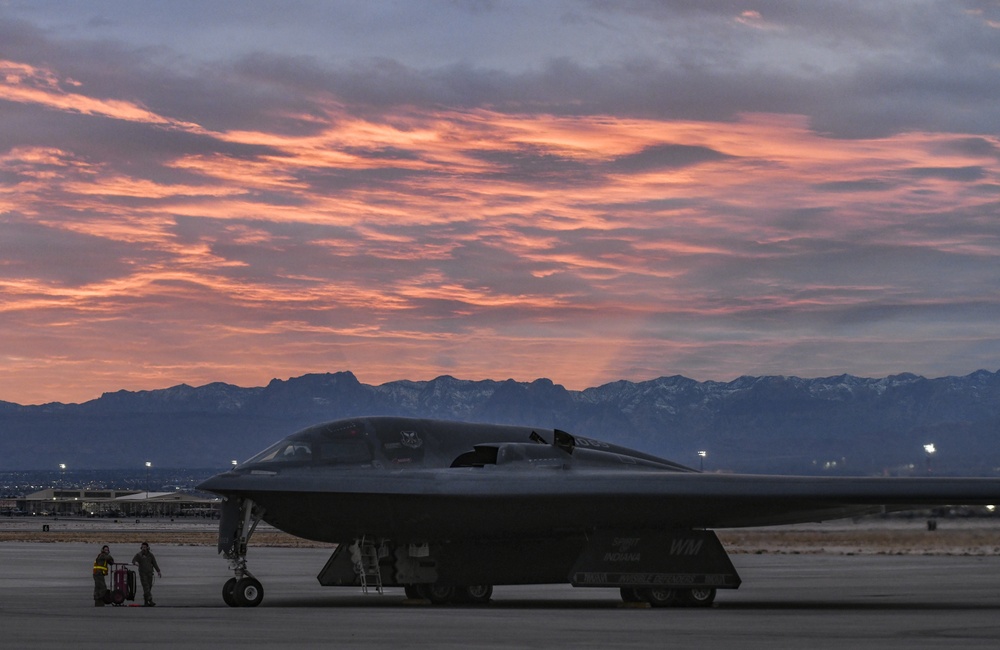The photograph, taken at dusk, captures an awe-inspiring scene featuring a sleek, black, and dark gray fighter jet prominently displayed on a runway. The twilight sky overhead is a stunning blend of pastel hues, including shades of pink, blue, gray, yellow, and orange, with bluest clouds shining through and light beams radiating from behind a distant mountain range. The mountains, tinged with white at their peaks, stretch evenly across the background, creating a majestic backdrop.

The fighter jet, with its distinctly smooth and rounded dome, large flat wings, and sleek profile, exudes a futuristic, almost alien appearance. The aircraft, marked with white lettering reading "Spirit of Indiana" and "WM" under its wing, faces the left of the image, captured in profile. The runway, part of what seems to be an airfield, includes light poles and distant buildings softly illuminated.

In the foreground, two workers in gray jumpers stand in front of the jet. The worker on the left wears a bright orange hazard vest while the worker on the right does not. They are accompanied by a white-framed, red metal trolley, adding to the authenticity and dynamism of this compelling twilight scene.